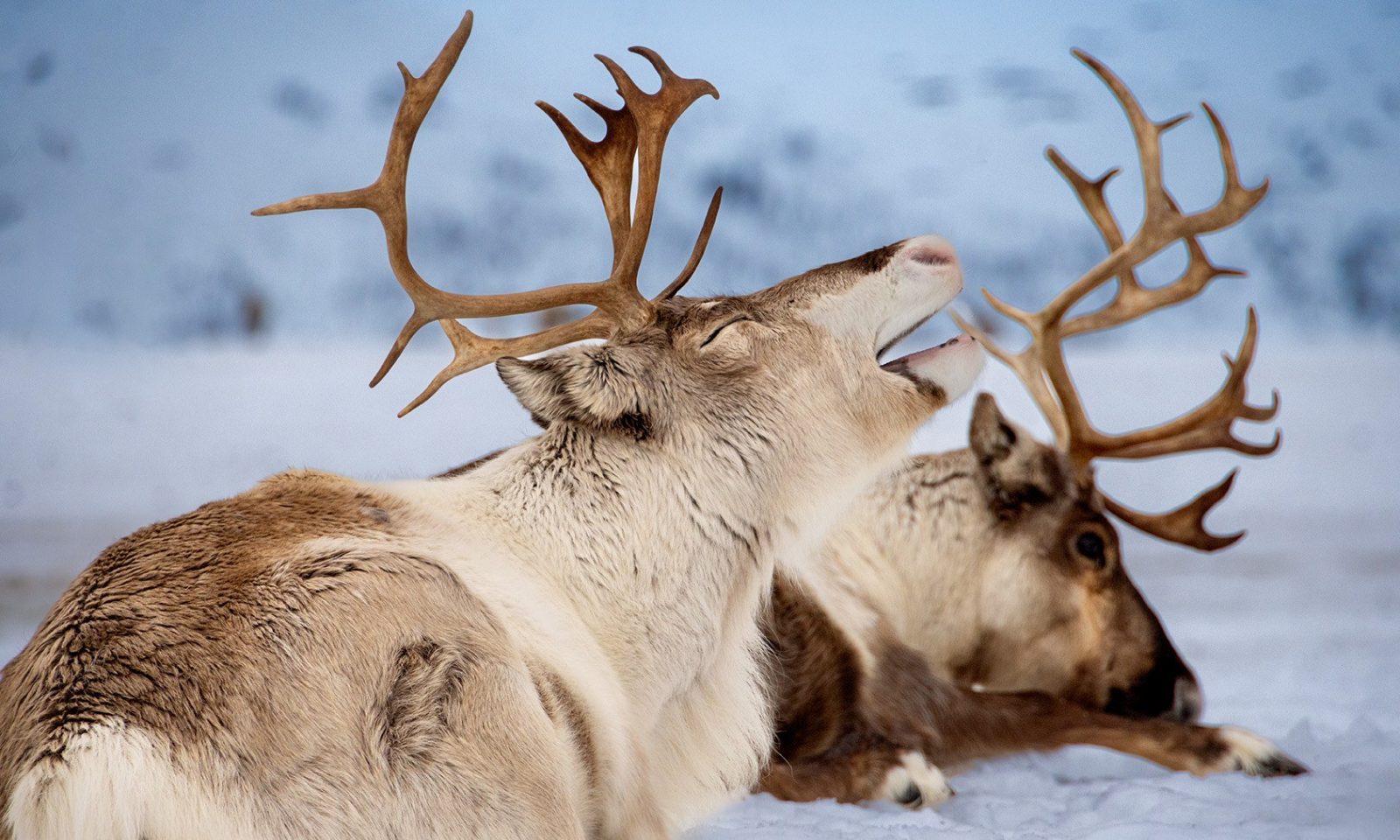The image showcases two reindeer resting on a snowy ground in a serene, cold climate. The background, though slightly blurred, appears to feature snow-covered trees, giving the scene a tranquil and frosty ambiance. The reindeer in the foreground displays a striking contrast in its coat, with a soft white and tan hue complemented by dark brown patches, particularly noticeable on its back. Its majestic brown antlers resemble tree branches, extending proudly from its head, which is lifted towards the sky, eyes closed, and mouth partially open as if calling out. Beside it, the second reindeer rests fully on the snow, with its head nestled on its foreleg and its antlers raised. This reindeer has a predominantly white top coat with dark brown and black shading on its back and legs, its dark nose almost touching the snow, and its eyes open, contrasting with the relaxed posture of its companion.